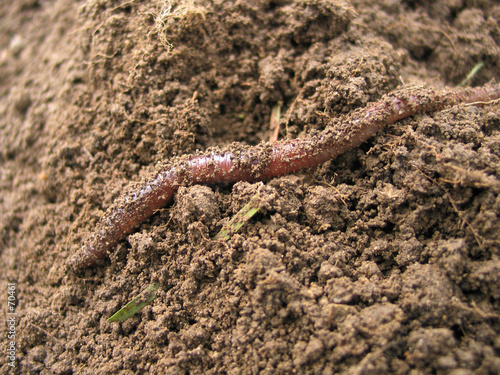This image is an extreme close-up or macro shot of a worm partially emerging from soft brown soil. The worm's body, covered in specks and clumps of dirt, stretches from the lower left to the upper right of the frame. It is difficult to determine which end is the head or the tail, but the worm's pinkish-reddish hue is visible beneath the dirt. The surrounding soil appears fine-grained and slightly sandy, with tiny roots, branches, and a piece of a leaf mixed in. The soil is dry, yet soft and loose, forming small valleys and "mountains" around the worm. There are no other significant elements in the frame, aside from some tiny, unrecognizable letters or numbers located in the lower left corner.